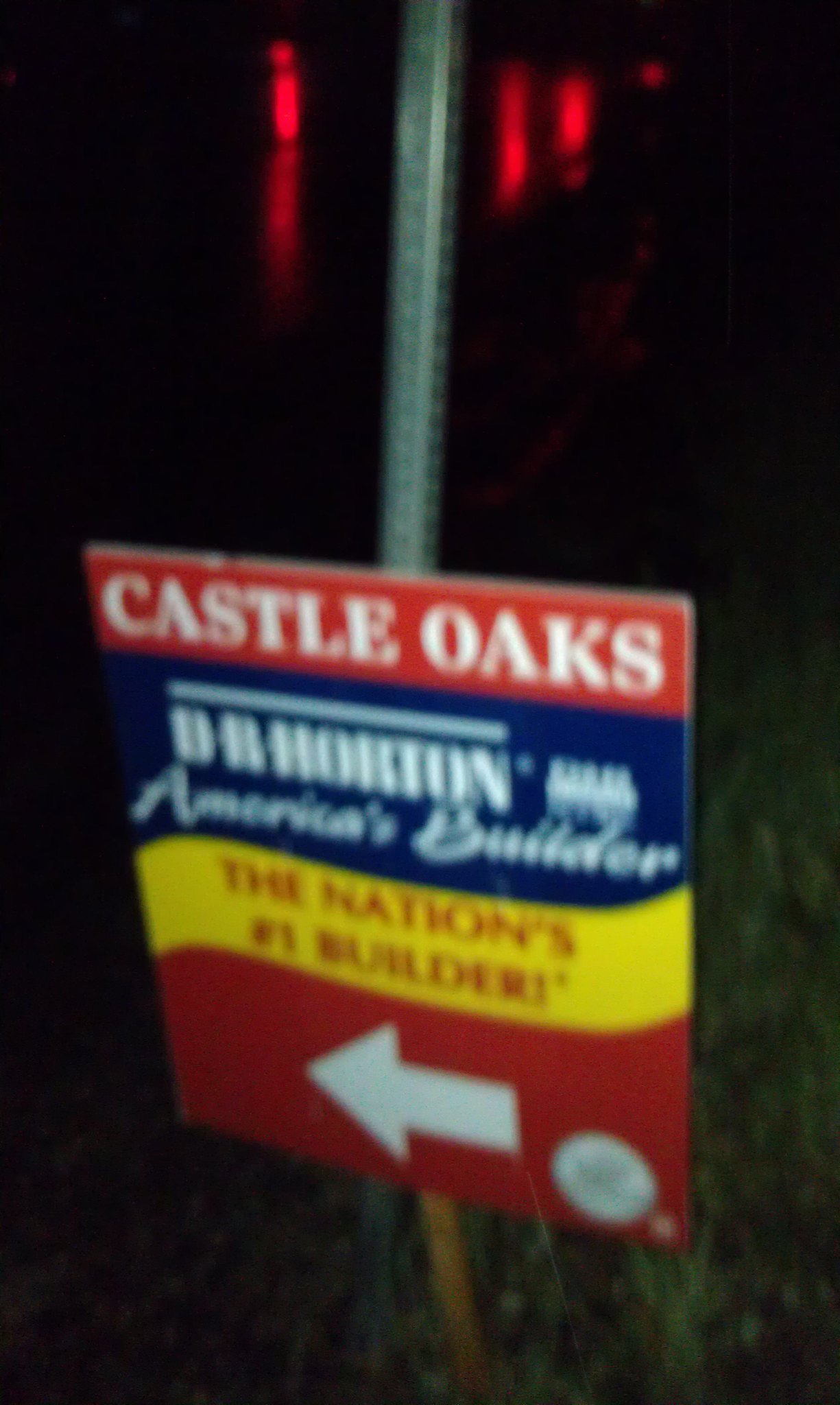In the blurry nighttime photo, illuminated solely by the camera's flash, a multicolored sign is mounted on a metal post and supported by a wooden stick. The sign, positioned in some grass and surrounded by green foliage, is an advertisement for a home builder. It sits in front of a grey pole, with some red lights visible in the distant background.

The sign's top section features a red rectangular banner with the text "Castle Oaks" in bold white capital letters. Directly below this, a blue banner spans the width of the sign, proclaiming "D.R. Horton, America's Builder" in white letters. Further down, a yellow banner with red letters announces, "The Nation's Number One Builder!" At the bottom of the sign, a large white arrow points to the left, set against a vibrant red background. Accompanying the arrow is a white circle, which serves as part of the company’s logo.